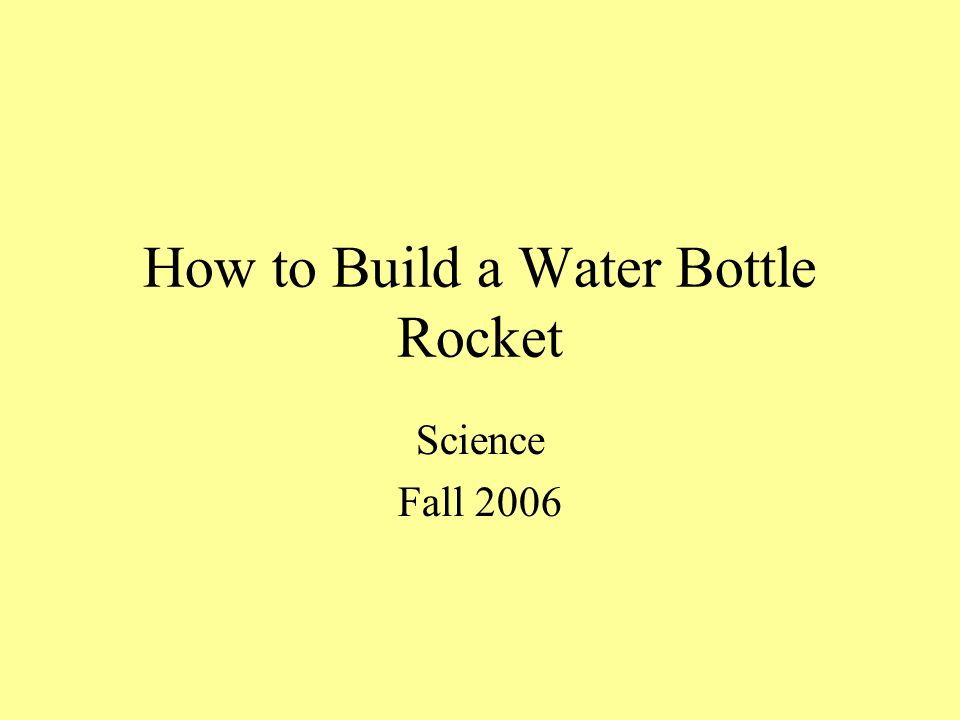The image is a square with a pastel yellow background featuring bold black letters. Centered at the top, it reads "How to Build a Water Bottle Rocket" with each significant word starting with a capital letter except for 'to'. Below this main title, there is a space, followed by the word "Science" also capitalized. Further down towards the bottom, it states "Fall 2006." The text appears to be laid out sequentially with "How to Build a Water Bottle" on the first line, "Rocket" directly below it, then a space followed by "Science" and "Fall 2006" in the lower section. The setting suggested by the design is possibly that of a school or library, indicating an educational or instructional context, possibly akin to a science project guide or a classroom poster.